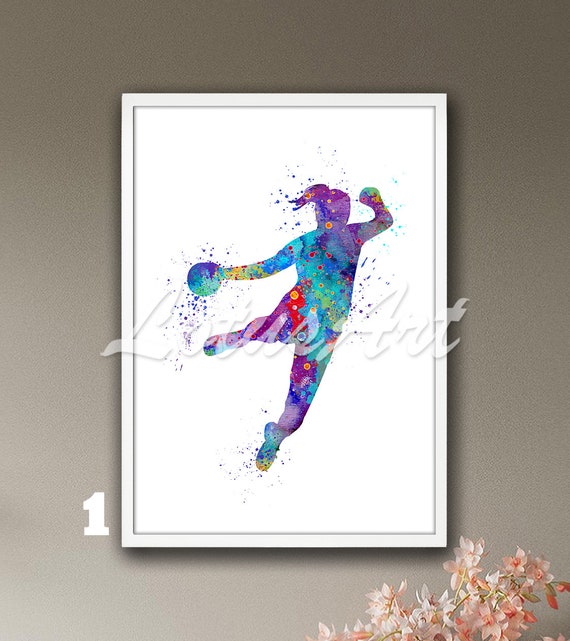This is an image of a colorful, abstract drawing of a woman with her hair pulled back in a ponytail. She appears to be engaged in a game, likely bowling, as she holds a ball in her left hand. Her right hand is extended backward, possibly holding another small, round object, and her right leg is raised in a dynamic pose. The woman's body is filled with an array of vibrant multicolors, including yellows, greens, purples, reds, and blues, arranged in stripes and mottled shapes. The background of the image is predominantly white, with a number "1" situated at the bottom left corner. The image also features some hard-to-read white text across it, potentially saying "Lotus Art." The drawing is encased in a white frame, and below the frame, the top part of pink flowers can be seen, adding a touch of natural ambiance to the overall composition.